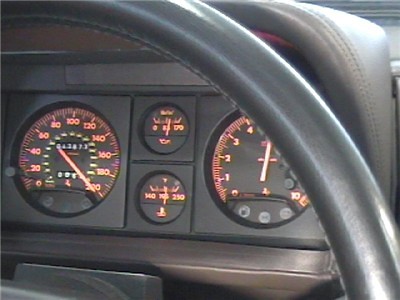The image captures the dashboard of an aged car, with the viewpoint looking through the classic gray leather steering wheel. The steering wheel itself spans from the top left to the bottom right of the frame, partially obscuring the view of the dashboard. This older model vehicle features a dashboard adorned with gray leather and complemented by gray paneling. Prominently displayed are four gauges: two large meters positioned on the far left and right of the dashboard, and two smaller meters situated one above the other in the center. All the meters are illuminated with a vivid neon orange hue. Light spills in from the top right corner, casting a glow across the dashboard and the upper section of the steering wheel. The rest of the steering wheel extends down to the bottom of the image. The photograph itself has a vintage quality, suggesting it was captured with an older camera, enhancing the nostalgic feel of the classic car.